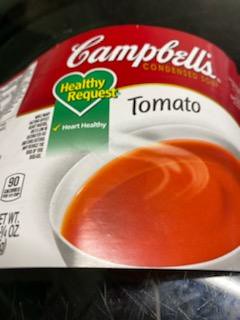A Campbell's soup label is displayed on a black granite or marble countertop, showcasing some noticeable scratch marks and a slight reflection of light in the bottom right corner. The label features the iconic Campbell's soup logo with a vibrant red border at the top, where "Campbell's" is written in white. Beneath this, the words "condensed soup" are printed in yellow, and a green "Healthy Request" heart logo with a check mark highlights the label's "heart healthy" claim. The label's white section contains the product name "tomato" in bold black print, along with "90 calories per serving" noted below. Adjacent to the text, there is a detailed image of a white ceramic bowl filled with rich red tomato soup, with wisps of steam rising to indicate its warmth and freshness.